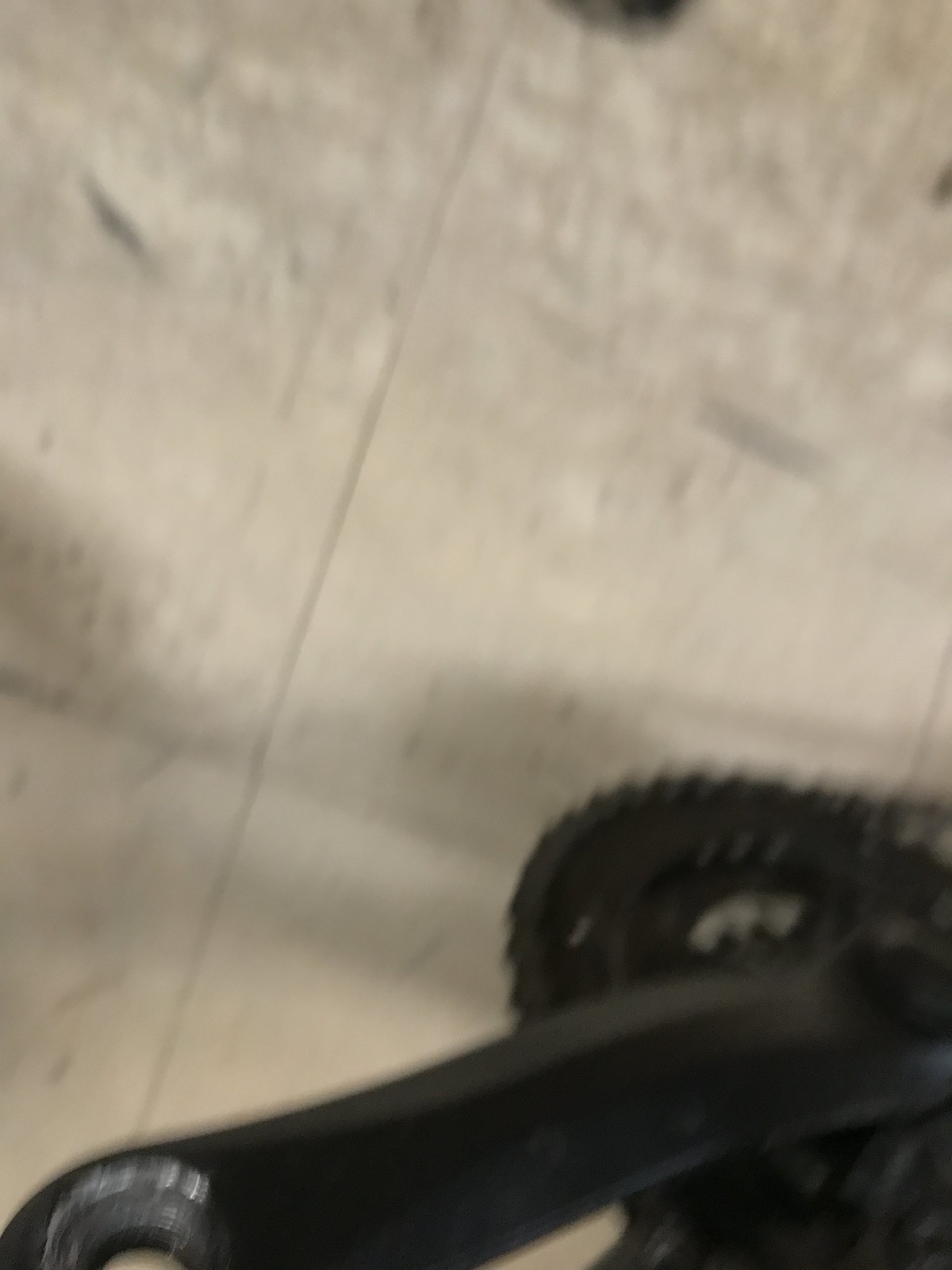This photograph provides an overhead view of a tool set against a white and gray mottled background. Located in the lower left-hand corner, the tool features a solid black metal handle that extends diagonally upward to the right, disappearing off the edge of the image about a quarter of the way up from the bottom. The handle, which has a rectangular shape, prominently displays a hole near its left end with a silver metal lining the inner edges. Additionally, a silver metal ridge outlines the top part of the hole. On the right side, the handle connects to a circular black metal component resembling a gear, complete with small metallic teeth along its edge, suggesting its function as part of a mechanical or industrial apparatus.